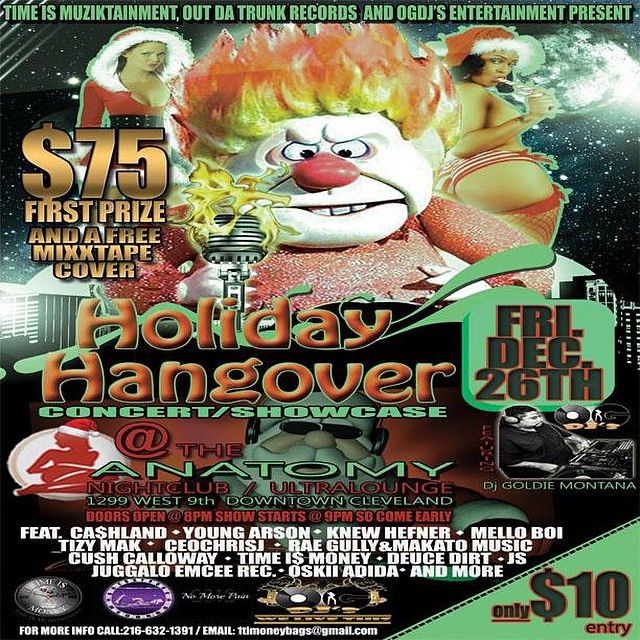The concert advertisement poster is vibrant and eye-catching, featuring an intense and detailed illustration. At the top, in bold green text, it reads: "Time, Musicainment, Outda Trunks Records, and Ogdee's Entertainment Presents." The central figure is an angry clown-like character with a white face, a red nose, and flames blazing from his head. He wears a red sparkly long-sleeved shirt. Flanking him on each side are scantily dressed women in festive, Christmas-themed outfits. The woman on his left sports a red suit with a white line accentuating her forehead and shoulders, resembling a sunny uniform. The lady on his right, with darker skin, bites a candy cane and wears red and white underpants along with white garments. She has black hair peeking out from a red and white cap and piercing brown eyes. 

Beneath the main illustration, there is a fiery microphone symbol and several text elements promoting the event. In vibrant orange, the title "Holiday Hangover" is displayed with green swishy lines behind it, followed by "Concert/Showcase." Further details include the venue, "The Anatomy, Nightclub/Ultra Lounge, 122 West 9th, Downtown Cleveland," with doors opening at 8 pm and the show starting at 9 pm. Attendees are urged to come early.

Additional information specifies a first prize of $75 and a free mixtape cover, highlighted under the left woman's image. Featured acts such as Cash Land, Young Arson, and New Hefner are listed, along with the entry fee of $10 noted in the lower corners. For further inquiries, contact details provided are a phone number (216-632-1391) and an email address (www.ttmonkeybags.gmail.com). The layout is busy yet festive, with green hues dominating the background, creating a lively and spirited visual.